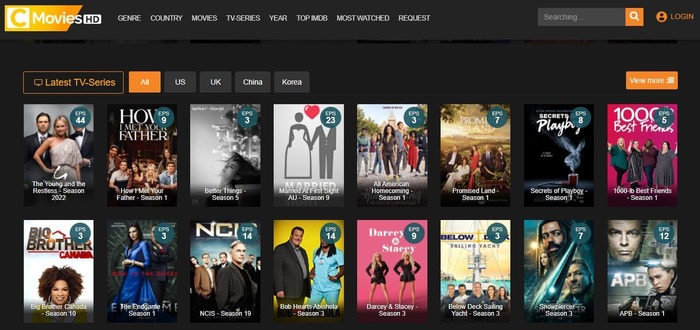The image portrays a computer screen displaying a streaming website with a predominantly black background. In the top left corner, there is a small yellow section featuring the label "AC" in a white box, followed by "Movies HD". To the right of this, a horizontal menu bar lists various navigation options: Country, Genre, Movies, TV Series, Year, Top Movies, Most Watched, and Request. On the far right side of this menu bar, there appears to be a search bar and a login option.

Below the menu bar, there are sections for browsing the latest TV shows, with filters for selecting content from the US, UK, China, and Korea. On the far right of this section, an orange "View More" button is prominently displayed. 

The main content of the screen comprises two rows, each containing eight thumbnails of TV shows. Each thumbnail includes the show’s title and an image representing the show. For instance, the first thumbnail in the top row is for "The Young and the Restless," featuring a promotional image with two men and a woman.